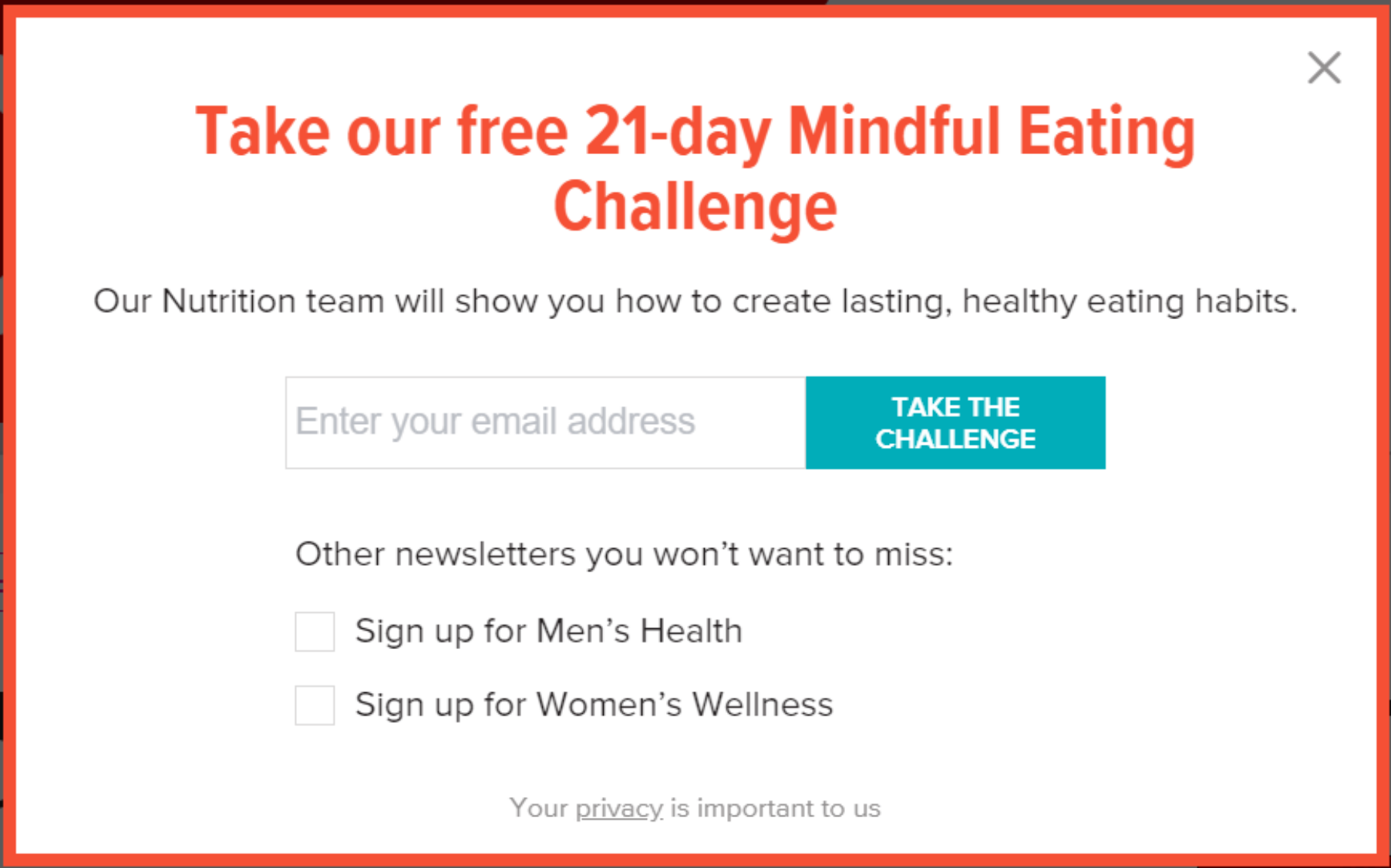In the image, a poster promotes a "Free 21-Day Mindful Eating Challenge," inviting participants to join the challenge to develop lasting healthy habits under the guidance of a nutrition team. Below the main text, there's a field labeled "Enter your email address," where users can input their email information. Adjacent to this field is an orange button labeled "Take the Challenge." Additionally, the poster offers options to sign up for newsletters with two checkboxes: "Sign up for Men's Health" and "Sign up for Women's Wellness," both of which are unchecked. The footer reassures that "Your privacy is important to us." The image is accented with an orange border, and some texts are highlighted in orange, while other elements are in green, black, and white. A close button is located at the top right corner of the image.